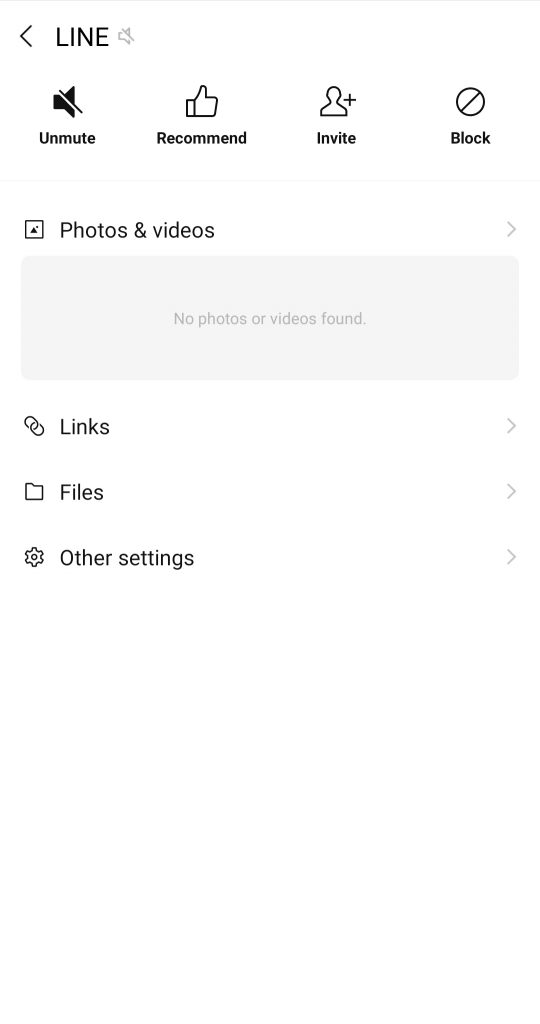### Caption:

This is a detailed view of a smartphone screen displaying various options related to a "Line" application. At the top of the screen, there is a back button on the left, followed by the word "LINE" in bold, all-caps black text. To the right of the text, there is a grayed-out speaker icon with a slash through it, indicating that the sound is muted.

Below this header, there are multiple menu options presented in list form. First is a black speaker icon with a slash through it, labeled "Unmute," which can presumably toggle the sound. Next to it, to the right, is a "Thumbs Up" icon labeled "Recommend." Following that is an icon of a person's outline with a plus sign, labeled "Invite," and finally, a circular icon with an angled slash through it, labeled "Block."

Further down, there is an icon depicting a triangle and a dot, resembling a mountain and sun inside a square, labeled "Photos and Videos." Adjacent to this is a gray "More" button. Beneath this, centered in gray text, are the words "No photos or videos found."

Continuing down, the interface shows two connected ovals labeled "Links," with another gray button to the right. Following that is a tabbed file folder icon labeled "Files," again with a gray button on the right. Below this, a gear icon is labeled "Other Settings" with another option next to it.

The remainder of the page is a large blank white space, indicating no further content or options are displayed on this screen.